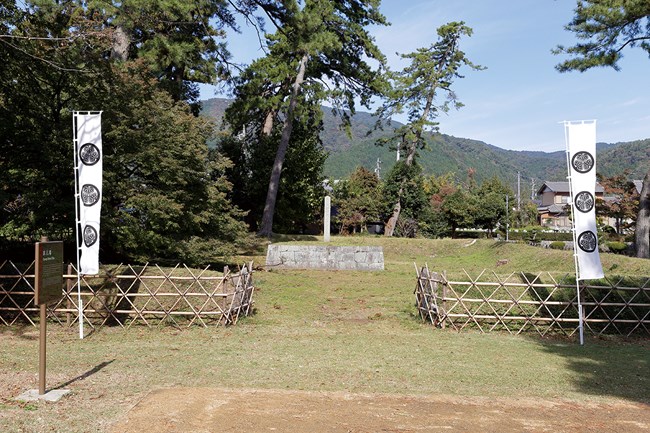The image captures an outdoor scene set in a natural environment featuring a variety of distinct elements. The foreground is dominated by a rectangular patch of bare red dirt, bordered by a three-rail wooden fence with crisscrossed uprights. An opening in the fence is flanked by tall white banners each adorned with three circular designs or logos. To the left, there's a brown interpretive sign on a post, though its text is not visible due to the angle. Behind the fence, a mix of evergreen trees and shrubs populate the scene, with a few buildings visible on the right. The background showcases mountains with green and gray tones, under a light blue sky streaked with small, feathery clouds. The ground outside the dirt patch is primarily grassy.